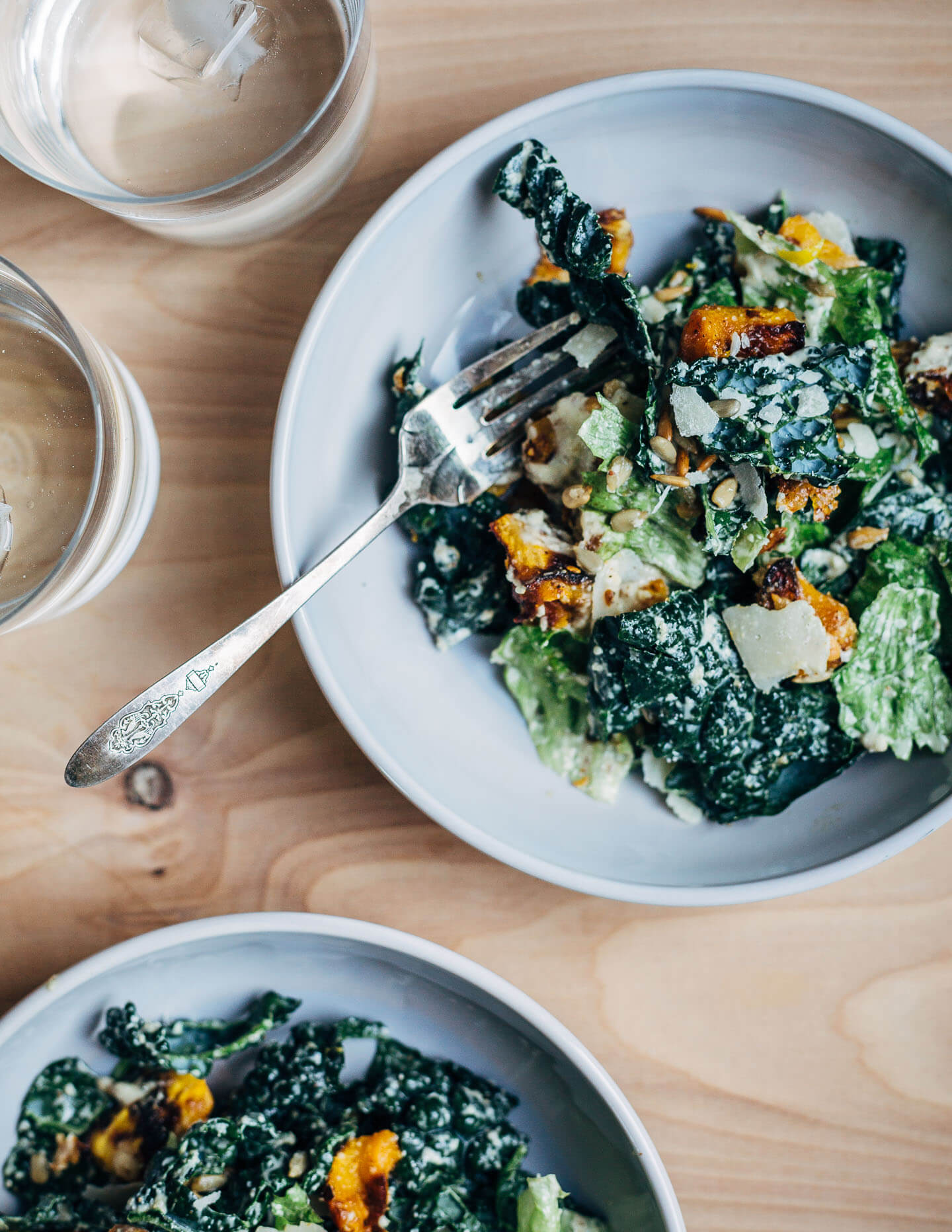The image features two healthy-looking salads presented in shallow, dark gray plastic bowls. Each salad is composed of vibrant sautéed greens, possibly fried or sautéed in a light oil, exhibiting a glistening, dark-green color. Among the greens, there's a mix of lean protein components, including chunks of chicken and perhaps pine nuts, identified by their small, grayish-brown appearance. Complementing the greens are orange-colored vegetables that look like seared squash or sweet potatoes, bearing distinct dark brown sear marks. In addition to these ingredients, the salads are topped with light green lettuce leaves and sprinkled with delicate flakes of Parmesan cheese, offering a light brown, crystallized texture.

These bowls are accompanied by silverware, specifically shiny metallic forks with designed handles, indicating a touch of elegance. The scene is set on a light brown wooden table, where the grains of the wood are visible, adding to the rustic feel of the image. Also present are two glasses of water, clear and filled with ice cubes, positioned to the left of the bowls. This top-down view captures the intricacies of a nutritious and appealing meal, emphasizing minimal heavy dressings in favor of high-quality ingredients.